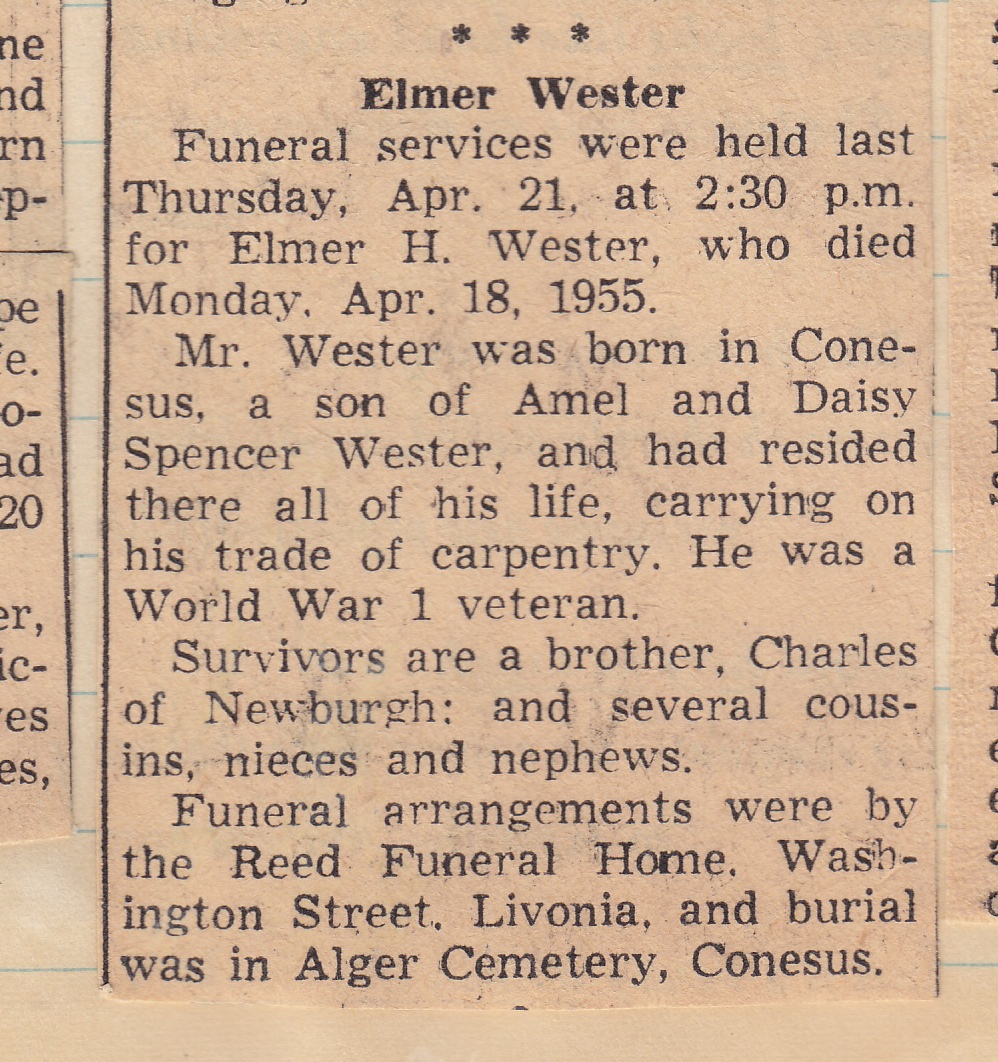This is an old, fragile, yellowed newspaper clipping with black writing, carefully cut out and placed on lined paper. The clipping, centered and weathered, is a funeral announcement for Elmer H. Wester, featuring bolded font at the top. The announcement reads: "Funeral services were held last Thursday, April 21st, at 2:30 p.m. for Elmer H. Wester, who died Monday, April 18th, 1955. Mr. Wester was born in Conesus, a son of Amel and Daisy Spencer Wester, and had resided there all his life, carrying on his trade of carpentry. He was a World War I veteran. Survivors are a brother, Charles of Newburgh, and several cousins, nieces, and nephews." Funeral arrangements were by the Reed Funeral Home, Washington Street, Livonia, and burial was in Alger Cemetery, Conesus.